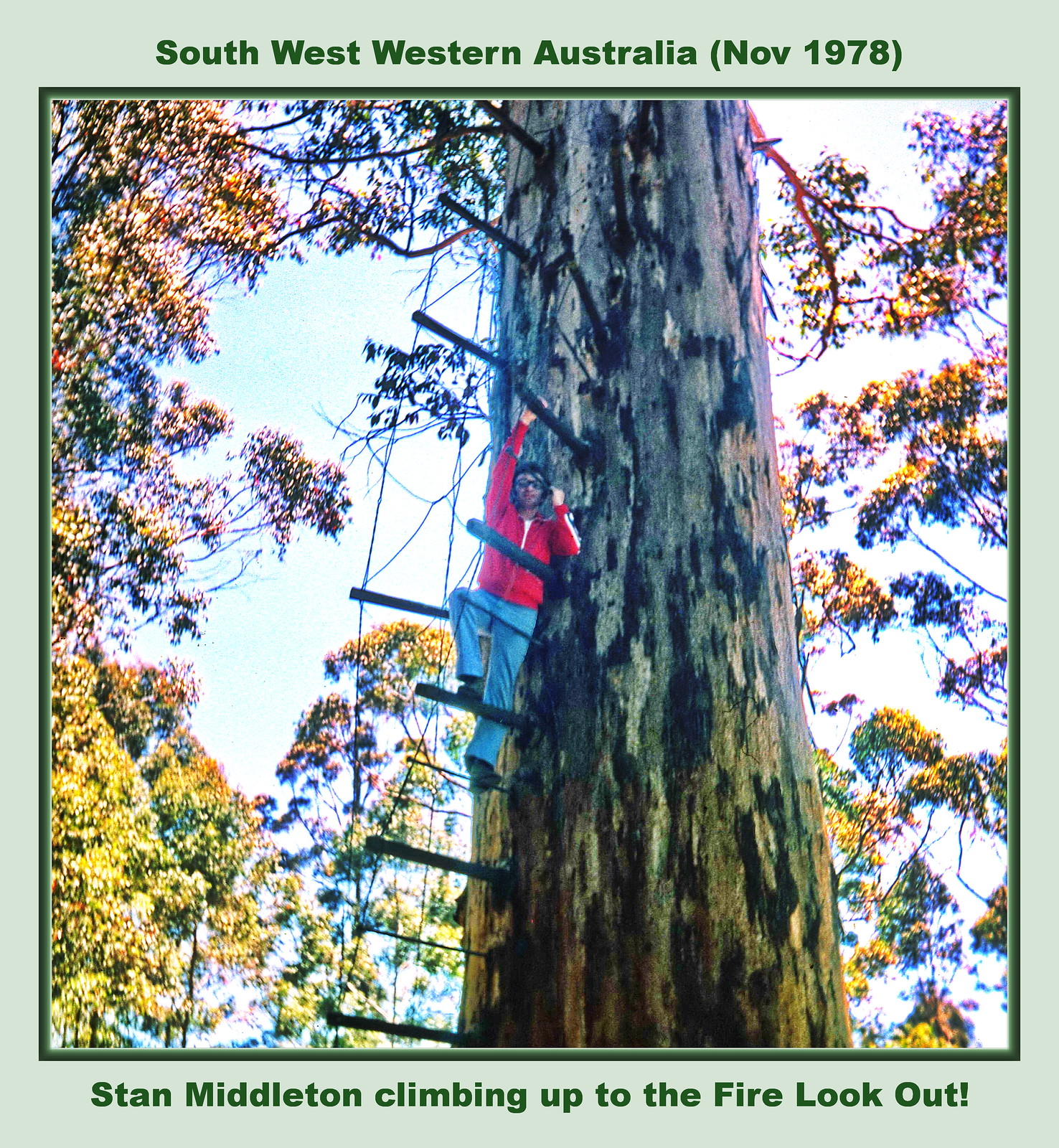The image is a color photograph surrounded by a light pastel green border with a dark green stripe on the top and bottom. At the top of the border, in green font, it reads "Southwest Western Australia (November 1978)" and at the bottom, "Stan Middleton climbing up to the fire lookout!" The photograph features Stan Middleton mid-climb on a giant tree trunk with extended spikes hammered into it, resembling a rudimentary fire lookout. He is wearing a red long-sleeve jacket and blue pants, and he has sunglasses on while he looks directly at the camera. His right hand grips one of the spikes, and his left hand is near his ear. The background is filled with colorful autumn leaves in shades of brown, purple, yellow, and some red, indicating it’s an autumn scene. The overall atmosphere is bright, suggesting it is daylight.